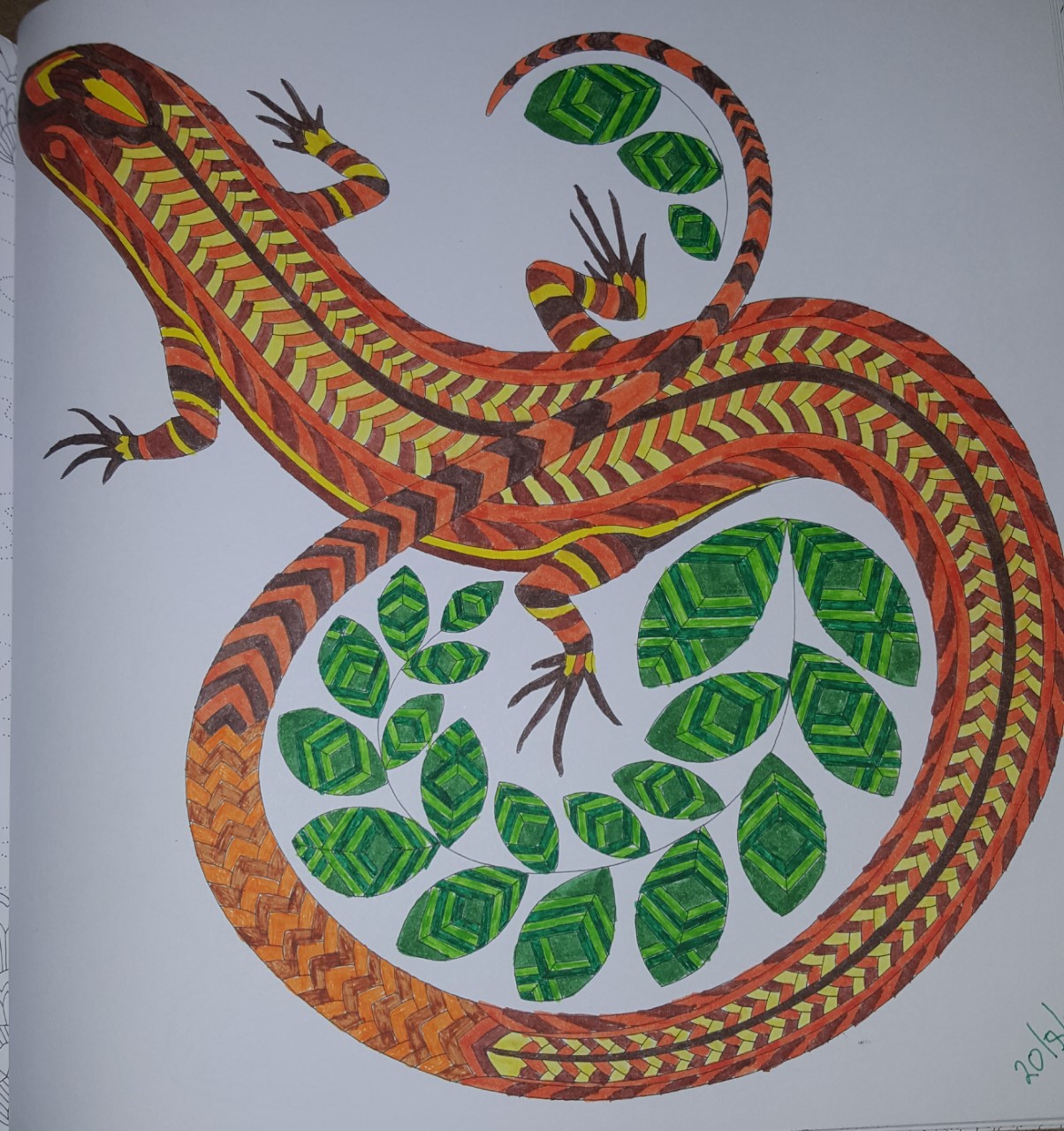The image displays a detailed drawing of a large, long-tailed lizard with a broad head, positioned on a white piece of paper. The lizard's head is situated in the upper left-hand corner, while its body extends down towards the center and then loops its tail in a circular motion that returns to the top-middle of the image. The creature is colored with a combination of dark red, reddish-brown, orange, yellow, and off-green hues. There is an orange stripe running down both sides of its body and a yellow stripe with black accents along the tail. The tail is notably longer than the lizard's body and features small brown v-shaped markings. 

The lizard's front limbs are depicted with almost human-like arms and five long fingers, whereas its back legs are shorter and more traditionally lizard-like. The background of the image includes multicolored green leaves with darker and lighter shades and some cleary discernible triangular or diamond-like patterns. These leaves are found both around the circle formed by the lizard's tail and at the tip of the tail. 

In the bottom right corner, there is a partially obscured date or signature that reads "2018" or "20-8."